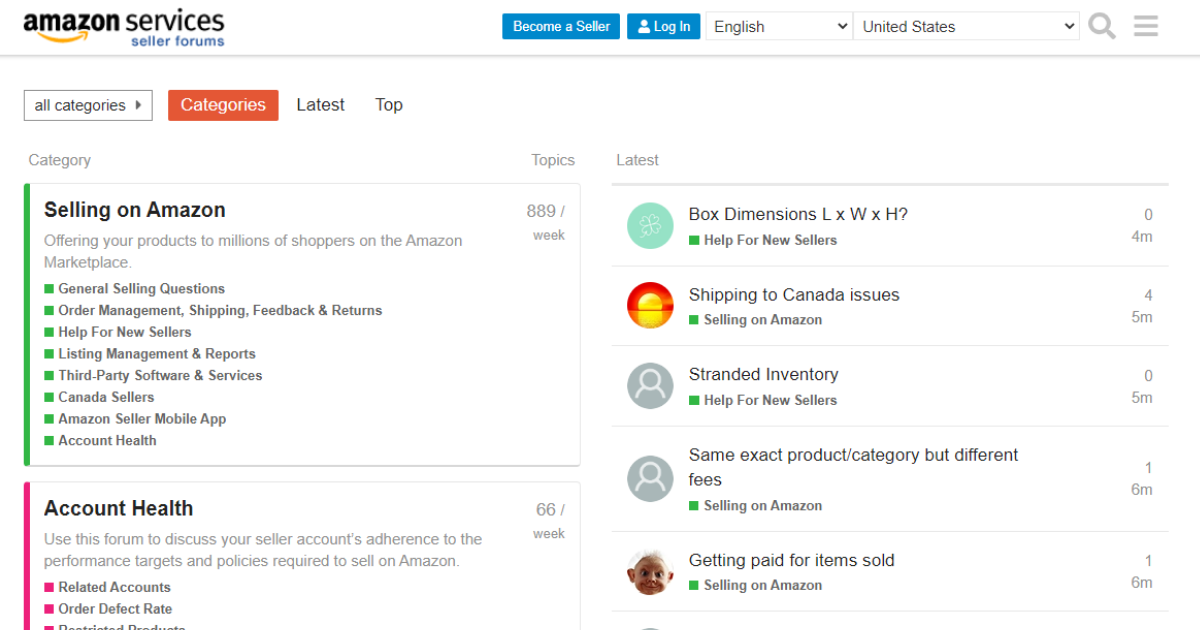This image features a white background dominated by the Amazon Services interface. At the top, the iconic Amazon logo is displayed, complete with its characteristic yellow arrow. Below this, two blue buttons are prominently visible: one labeled "Become a Seller" and the other "Log In". 

There is also a language selection box indicating "English" with a downward arrow, and a location setting for the "United States" with another downward arrow next to it. Nearby are icons including a magnifying glass and three horizontal lines, typically indicating a search function and menu respectively.

A horizontal blue line serves as a separator, under which a dropdown box reads "All Categories". Next to it, there's a red box labeled "Categories" and a navigation bar featuring tabs such as "Latest" and "Top".

The main content section is introduced by the titles "Category Topics" and "Latest". The first highlighted box has a green vertical line on the left and the header "Selling on Amazon: Offering your products to millions of shoppers on the Amazon marketplace," denoted with "889/week". Various points under this header have green boxes beside them indicating different topics like "General Selling Questions".

Following this, a second box features a pink vertical line and the title "Account Health", marked with "60/week" in the top right. Each point associated with this section has a pink square, encompassing topics such as "Order Defect Rate".

To the right, under the "Latest" section, several blue-highlighted entries are visible. Topics include:
- "Box Dimensions: L × W × H?" with a small green box for "Help for New Sellers" and an activity metric of "0/4M".
- "Shipping to Canada Issues" marked with "Selling on Amazon" and "4/5M".
- "Stranded Inventory", also under "Help for New Sellers" with "0/5M".
- "Same Exact Product Category but Different Fees", under "Selling on Amazon" labeled "1/6M".
- "Getting Paid for Items Sold", once again under "Selling on Amazon" noted as "1/6M".

Overall, the image provides a detailed look into the user interface for Amazon Seller Forums, highlighting a variety of tools and resources available to sellers.